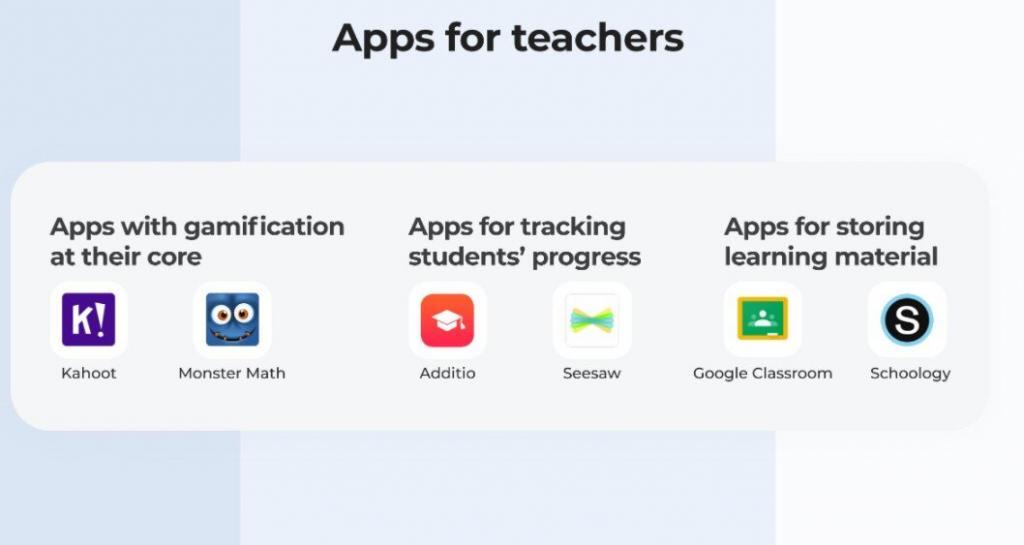A detailed screenshot features a layout of three vertical rectangles arranged side by side. The first rectangle on the left is blue, the middle one is light blue, and the third one on the right is a very light gray. Superimposed across all three rectangles is a translucent gray overlay. 

In the middle light blue rectangle, there is a collection of app icons tailored for teachers. At the top, prominently displayed, is a purple square with a white "K" and an exclamation mark, representing the app "Kahoot!". Beside it is a blue icon featuring a cartoonish monster face known as "Monster Math", indicating its gamified nature. 

Further down, the layout includes an orange square with a white mortarboard icon, symbolizing educational applications that track student progress. Additionally, there is an app with a teal addition symbol and a white square with a green bow-tie, identified as "Seesaw". 

Lastly, applications for storing learning material are showcased. This includes a green chalkboard icon for "Google Classroom", and a white square with a black circle containing a white "S" for the app "Schoolology".